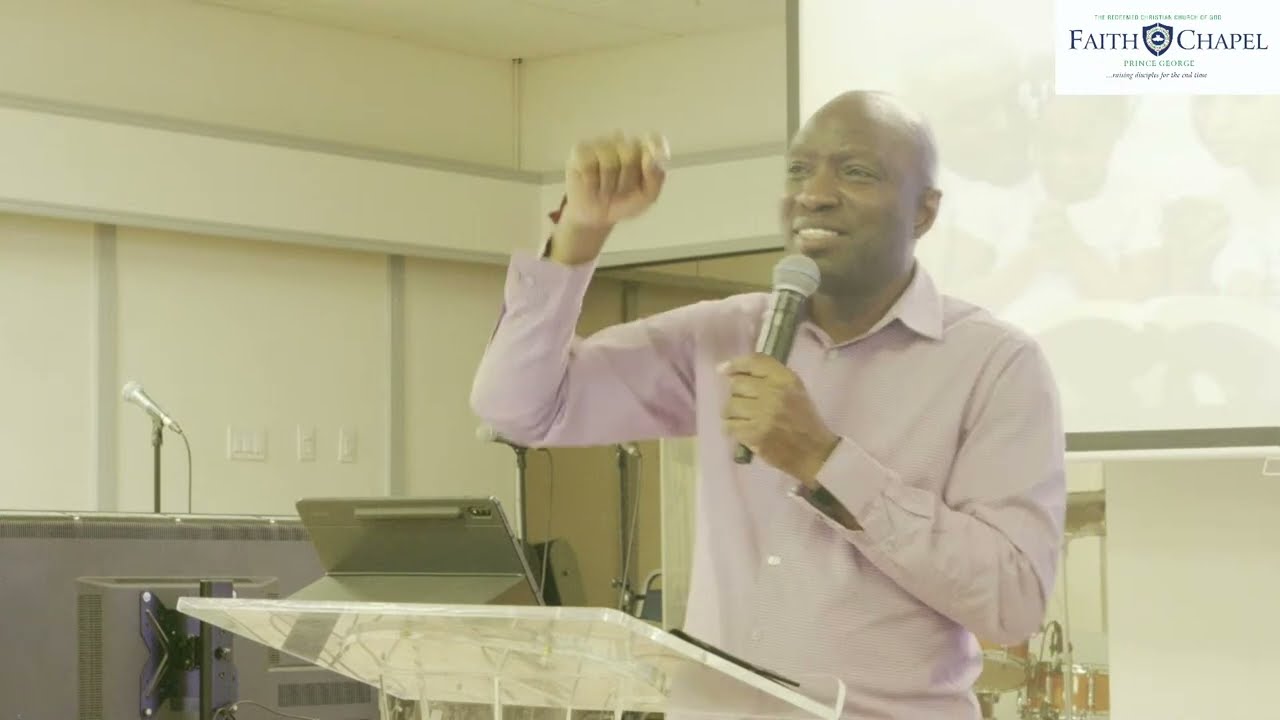The image depicts a black man, possibly a pastor, delivering a speech or sermon at Faith Chapel in Prince George. He is standing behind a clear lucite podium, with an iPad placed on it. The man is bald and dressed in a long-sleeved pink collared shirt with pearlescent buttons. His left hand holds a microphone up to his mouth while his right hand is raised, clenched in a fist, with his arm bent at the elbow. He is smiling, revealing his upper row of teeth, and is looking out at the crowd. Behind him, a projection screen is visible, displaying the "Faith Chapel" logo in blue font in the upper right corner. Additionally, a drum kit is partially visible in the lower right corner of the image, and to the left, there is another microphone stand with no one in front of it. The scene is well-lit, and the photograph captures various elements indicating that this is likely a church service or presentation.